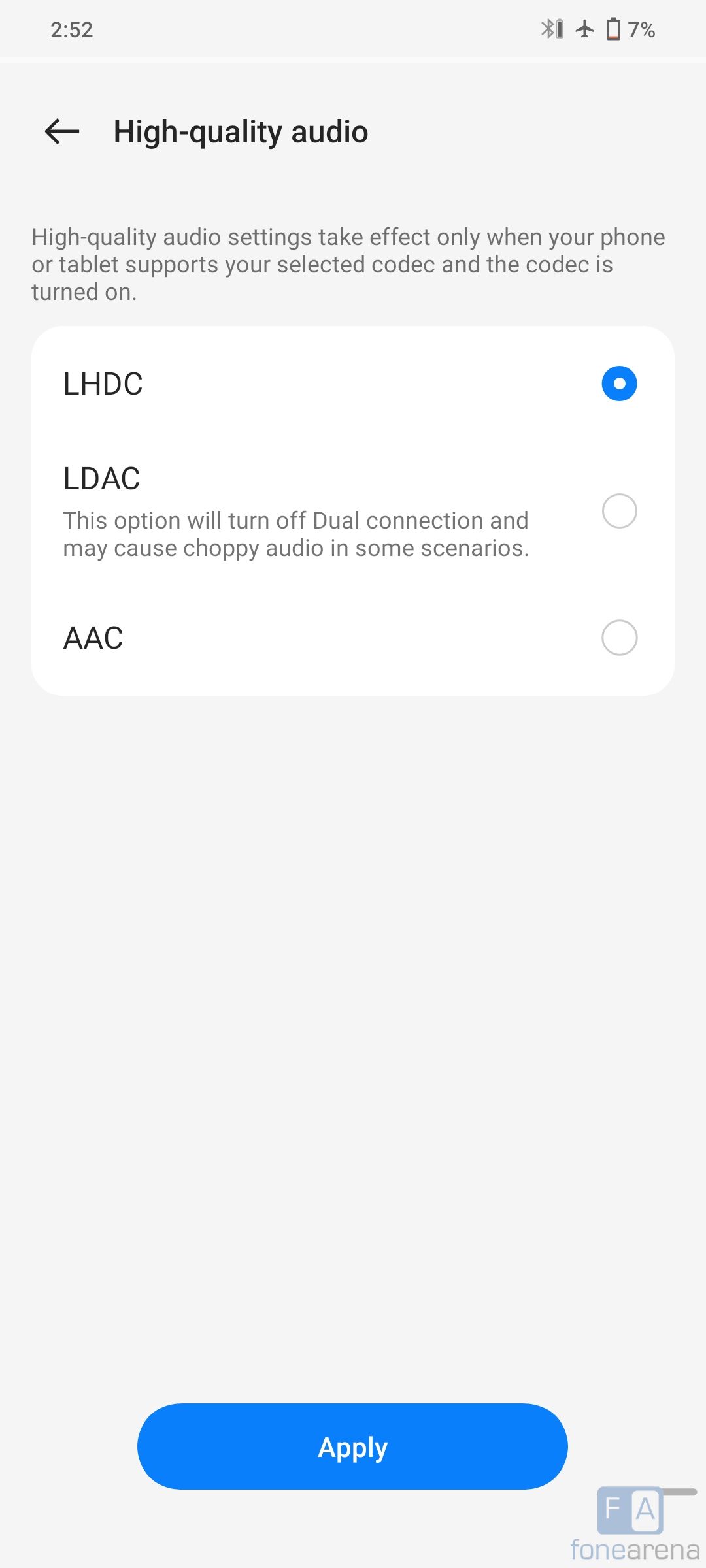The image is a screenshot taken from a smartphone in light mode. At the top, the status bar shows the time "2:52" in black, alongside icons for Bluetooth, airplane mode, and a battery indicator displaying 7% charge. 

Dominating the center of the screenshot is a header in bold black letters that reads "High Quality Audio." Below this header, there are three lines of text explaining the functionality: "High quality audio settings take effect only when your phone or tablet supports your selected codec and the codec is turned on."

Directly underneath this explanation is a white rectangular selection box with three codec options. Each option is accompanied by a circular selection button:

1. "LHDC" - This option is selected, indicated by a blue filled circle.
2. "LDAC" - This option is not selected. A note underneath specifies, "This option will turn off dual connection and may cause choppy audio in some scenarios."
3. "AAC" - This option is also not selected.

At the bottom of the screen, there is a prominent blue elliptical button with the word "Apply" inscribed in white letters.